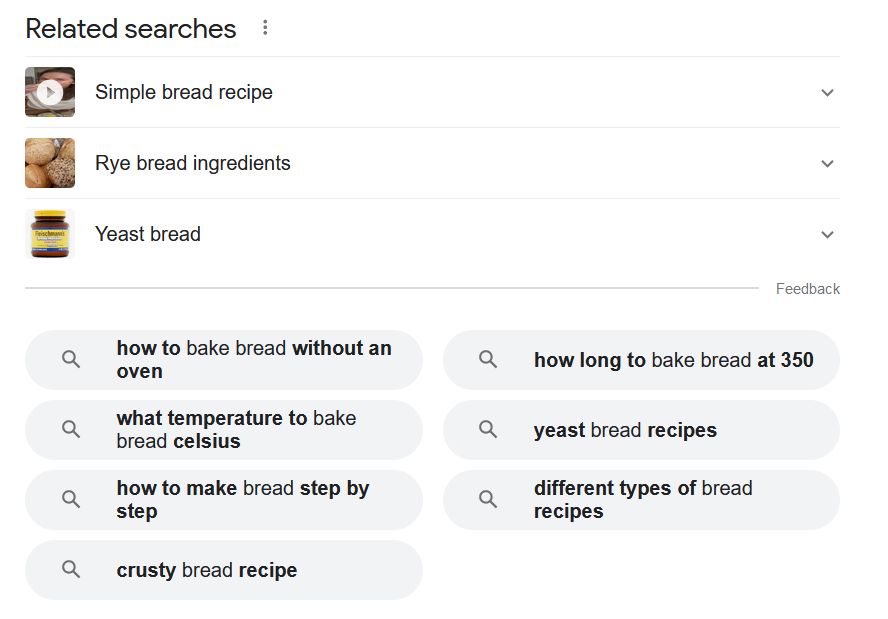This screenshot from a web page features a "Related Searches" section at the top, against a clean white background. To the right of the "Related Searches" title, there are three vertical dots indicating additional options. Immediately below this line, the section showcases three main entries with corresponding visuals and dropdown arrows on the far right for further interaction.

The first entry includes a video logo with the text "Simple Bread Recipe" next to it, followed by a downward-pointing arrow for a dropdown menu. The second entry presents an image of rye bread accompanied by the text "Rye Bread Ingredients" and another dropdown arrow. The third entry displays a picture of Fleischmann's yeast with the label "Yeast Bread" and a similar dropdown arrow on the far right.

Beneath these entries, there is a list of search recommendations, each presented within gray bars on the same white background. Each bar is marked with a magnifying glass icon on the left, indicating clickable search queries. The suggestions progress as follows:

1. "How to bake bread without an oven"
2. "How long to bake bread at 350"
3. "What temperature to bake bread Celsius"
4. "Yeast bread recipes"
5. "How to make bread step by step"
6. "Different types of bread recipes"
7. "Crusty bread recipe"

This layout effectively organizes related search topics, providing users with a variety of options for further bread-related inquiries.